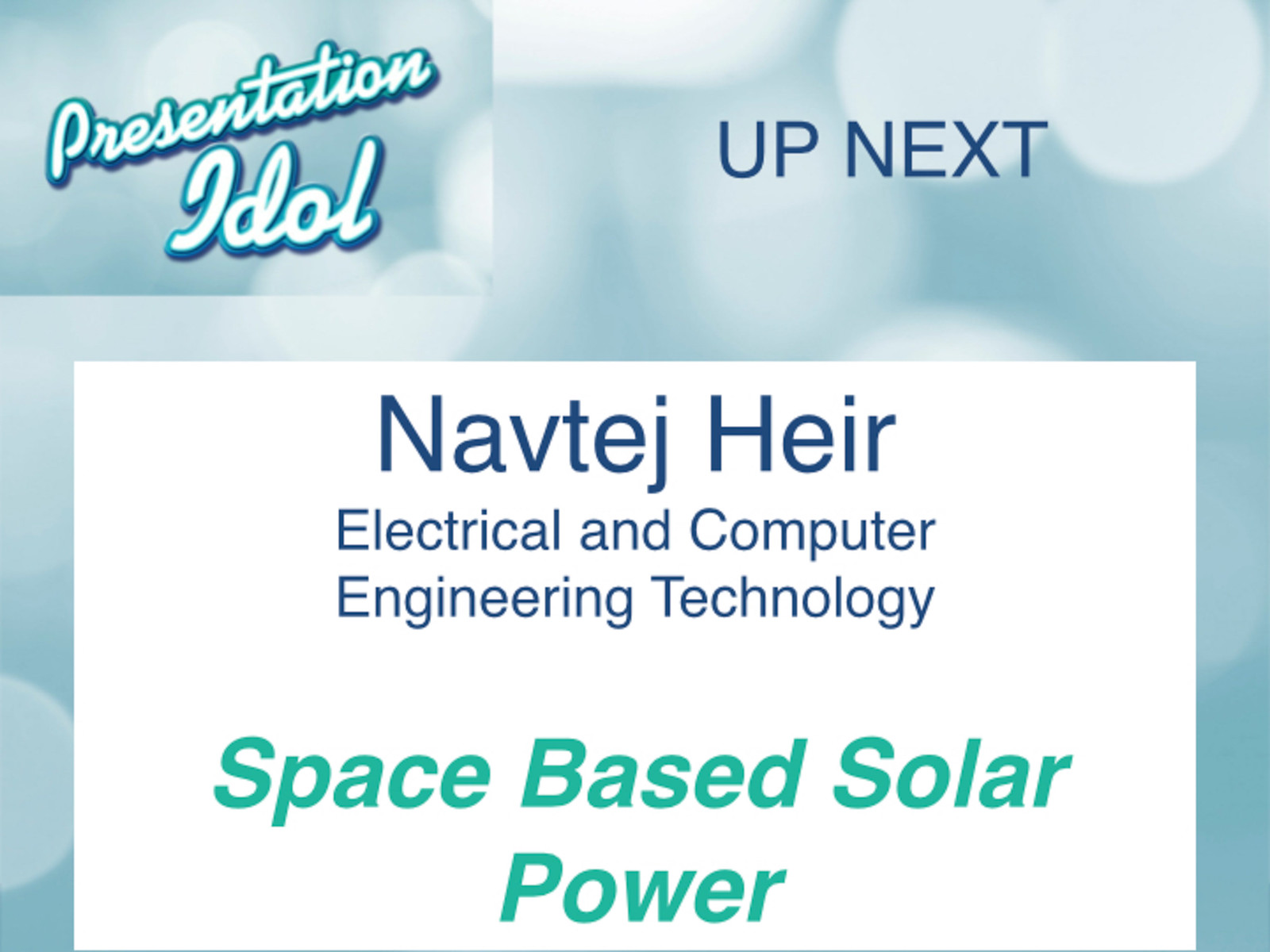The image shows a slide from a presentation with a light blue background interspersed with whitish-blue spots. In the top right corner, it reads "UP NEXT" in dark blue, all caps. The top left corner features a patchwork-like cutout that says "PRESENTATION IDLE" in a cursive font. The bottom half of the slide contains a prominent white text box. This box displays the name "NAVJEJ" followed by "ELECTRICAL AND COMPUTER ENGINEERING TECHNOLOGY" beneath it, all in blue text that aligns nicely in two lines. Below this, in green text on separate lines, it reads "SPACE-BASED" and "SOLAR POWER." The overall design suggests it is an introductory slide for a presentation titled "Space-Based Solar Power" by Navtej from the Electrical and Computer Engineering Technology department. The background has a blurred, bubble-like texture, giving it a subtle and modern look.